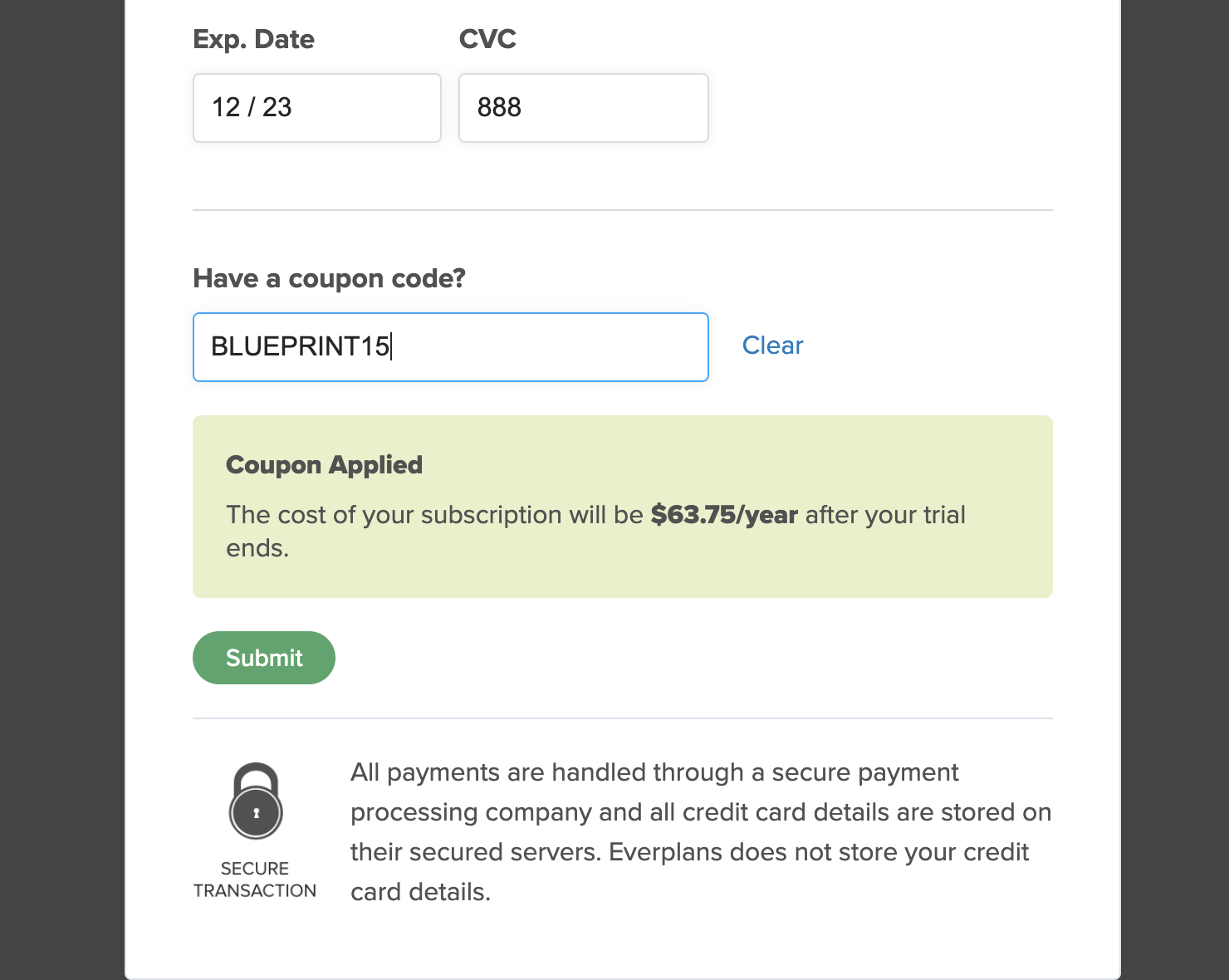The image depicts a pop-up interface for entering payment information, including coupon details, on a subscription service website. The sides of the pop-up are black, framing a white central section. At the top, there is a field labeled "Expiration" or "Exp. Date," with the sample input "12/23." Below it, another field is labeled "CVC," with a placeholder input of "888."

There is also a section for entering a coupon code, displaying the text "Have a coupon?" The data field for the coupon code has a white background with a blue outline and contains "BLUEPRINT15" in all capital letters. To the right of this field, there is a green rectangle displaying the text "Coupon Applied."

Additional details specify that the cost of the subscription will be $63.75 per year after the trial period ends. A green "Submit" button with white text is located on the left side. Beneath this, the pop-up includes a security statement asserting that the transaction is secure, symbolized by a keyhole icon. It states that all payments are processed through a secure company and that EverPlans does not store credit card details. The majority of the background is white, with green highlights indicating active fields and buttons.